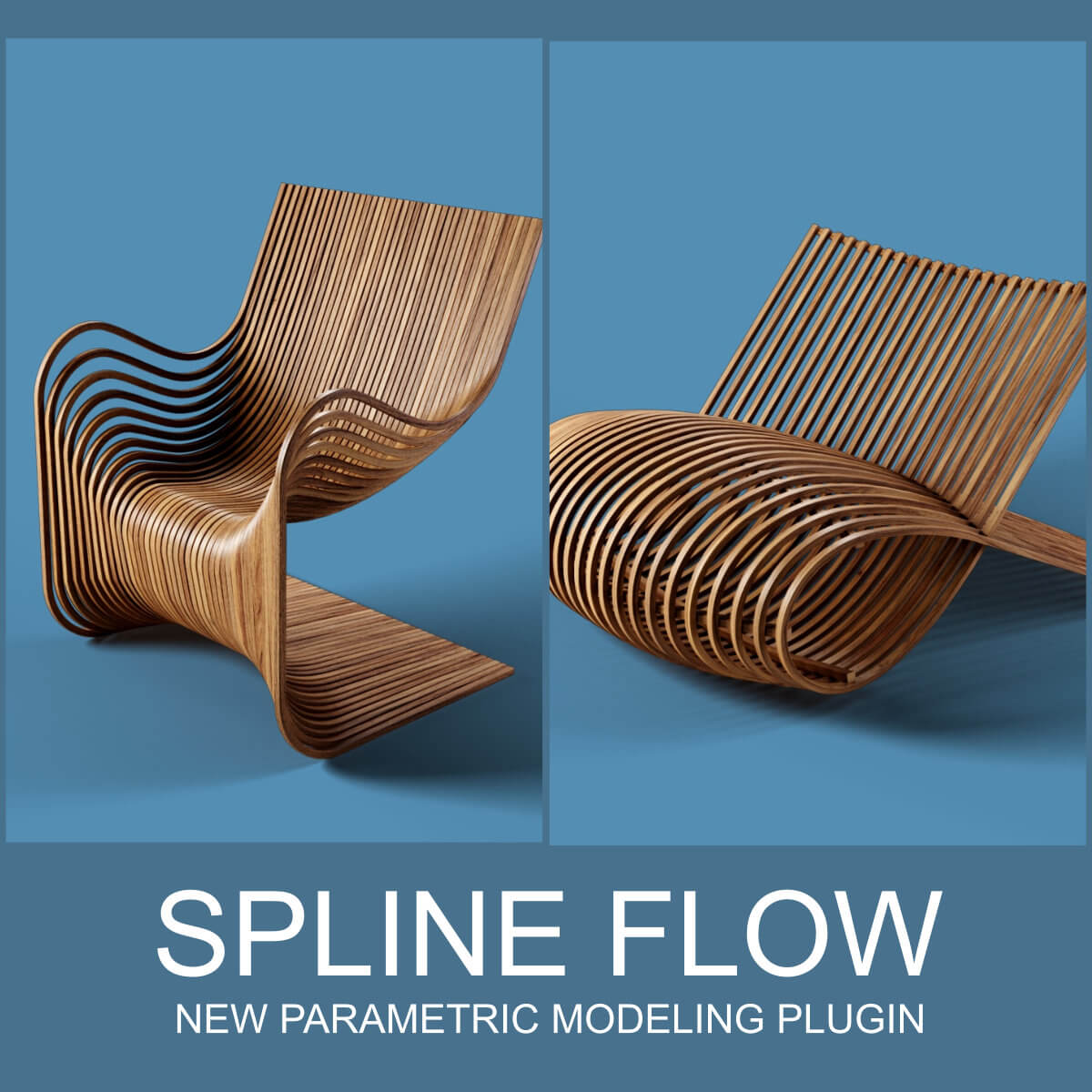The image contains two distinct chair designs made of rattan, illustrating the capabilities of the "Dual Parametric Modeling Plug-in" labeled as "Spline Flow." The chair on the left showcases a traditional shape with intricate rattan lines, featuring armrests and a curved seating area. In contrast, the right chair, devoid of arms, displays a unique design where the seat curves downward to seamlessly form the base. Both designs emphasize flexibility and curvature, demonstrating the potential for innovative, adjustable furniture structures using the parametric modeling plug-in described at the bottom of the image. The chairs' warped and wavy appearances suggest an exploration into dynamic and modular design possibilities.